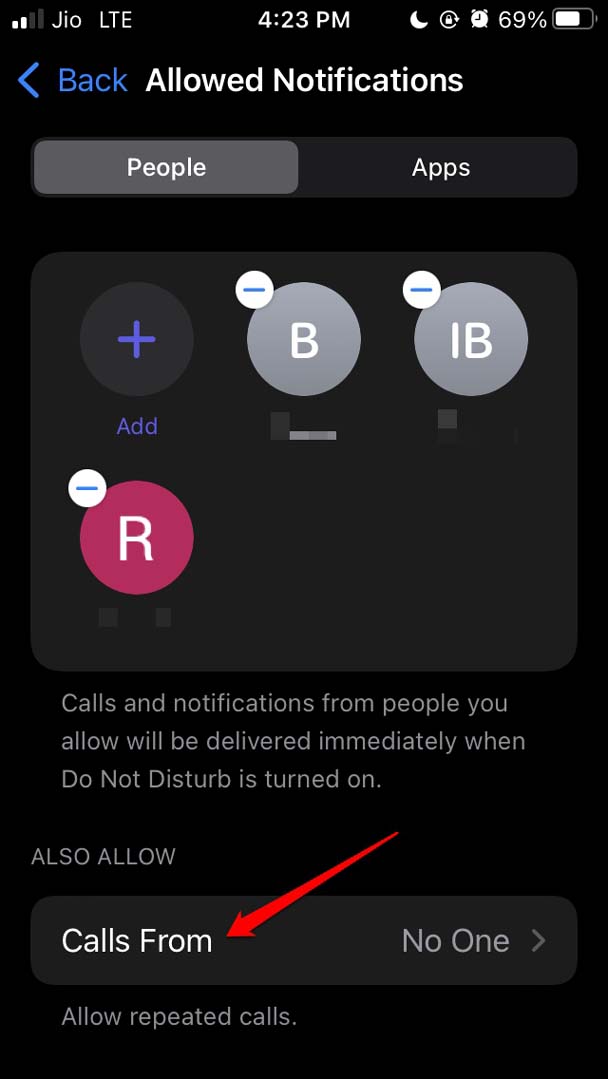Here is the detailed cleaned-up caption:

---

The image showcases a vertical screenshot of a mobile application, which seems to be designed for a smartphone or tablet. The app interface features a black background with text primarily in white and gray, and some elements in blue. At the top of the screen, the device status bar is visible, showing the network label "JIOLTE" on the left, the time "4:23 p.m." in the center, and various icons on the right, including a moon icon, an alarm icon, and a battery icon, all in white.

Beneath the status bar, the header indicates the title "Allowed Notifications" in white text. To the left of this header is a back button labeled "Back" in blue text. Below the header, there are two clickable option buttons: "People" and "Apps." The "People" option is selected, highlighted by a gray box, while the "Apps" button remains unselected in black.

Under these options, the screen displays four circular icons, arranged with three in the first row and one in the second. These circles are labeled with a plus symbol (+), the letters "B" and "IB," and the letter "R," respectively. Each of these circles has a minus sign next to it, indicating the ability to rearrange or modify the items.

Further down, the text explains the function: "Calls and notifications from people you allow will be delivered immediately when Do Not Disturb is turned on." Below this message, there is an option marked by a red arrow, labeled "Also allow calls from," followed by "Calls from" and the selection "No one."

---

This new caption provides a detailed description of the app's interface, making it easy to visualize the screenshot.